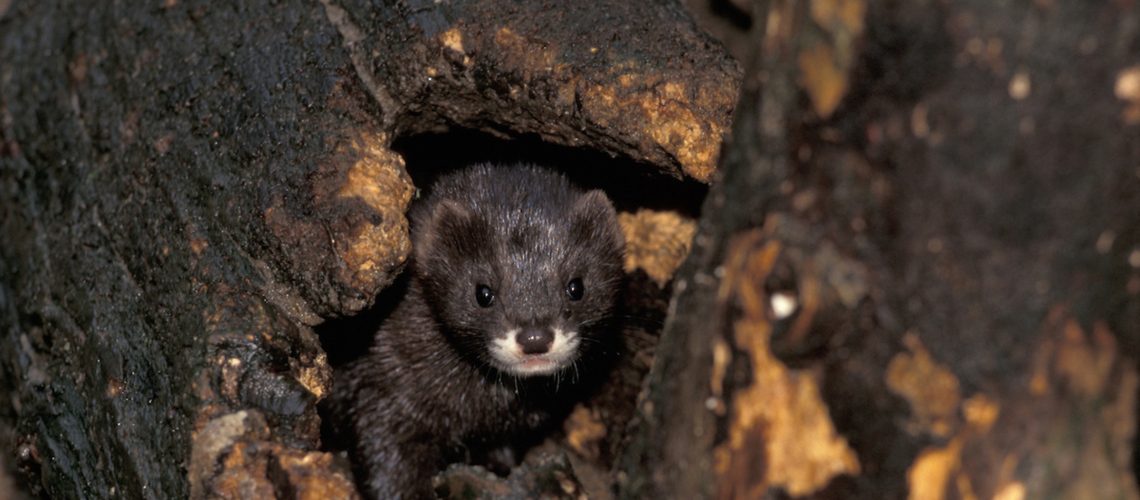In this photograph, a small rodent-like creature, possibly a weasel or ferret, peers out from the hollowed, darkened trunk of a fallen tree. The animal, which has a dark brown coat, beady eyes, and small pointed ears, gazes directly into the camera with a tiny brown nose and a white mouth framed by gray whiskers. The scene is set against a backdrop of a wet, rotted tree root that forms a black hole from which the creature emerges. Another dead, upright tree trunk, blackened with age and moisture, stands in the foreground. The overall setting is earthy and natural, highlighting the animal's curious yet cautious demeanor.